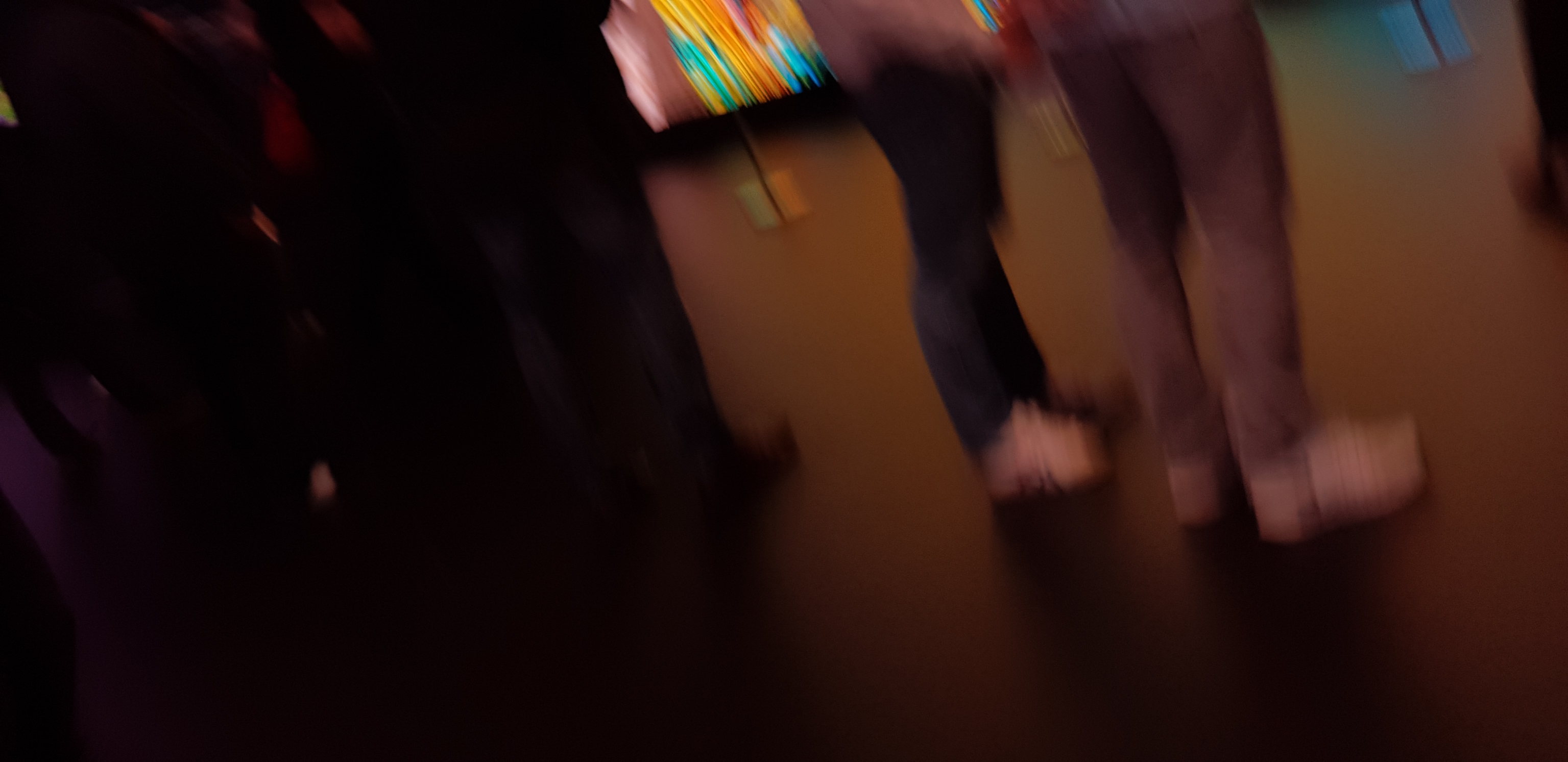The image captures a dimly lit setting, focusing primarily on the legs of two individuals standing side by side. The person on the left is clad in blue jeans, while the person on the right sports darker pants, nearly black, made from a similar denim fabric. Both individuals are wearing light-colored shoes. The ground beneath them is a dark surface, seemingly reddish due to the ambient lighting reflecting off it. In the background, a blurry array of lights in hues of yellow, red, blue, and orange create an abstract backdrop, suggestive of a poster or signage further inside the room. The setting includes dark, indistinct edges of large objects or partitions, yet the image is tightly cropped to emphasize the lower half of these figures amidst the ambient glow.